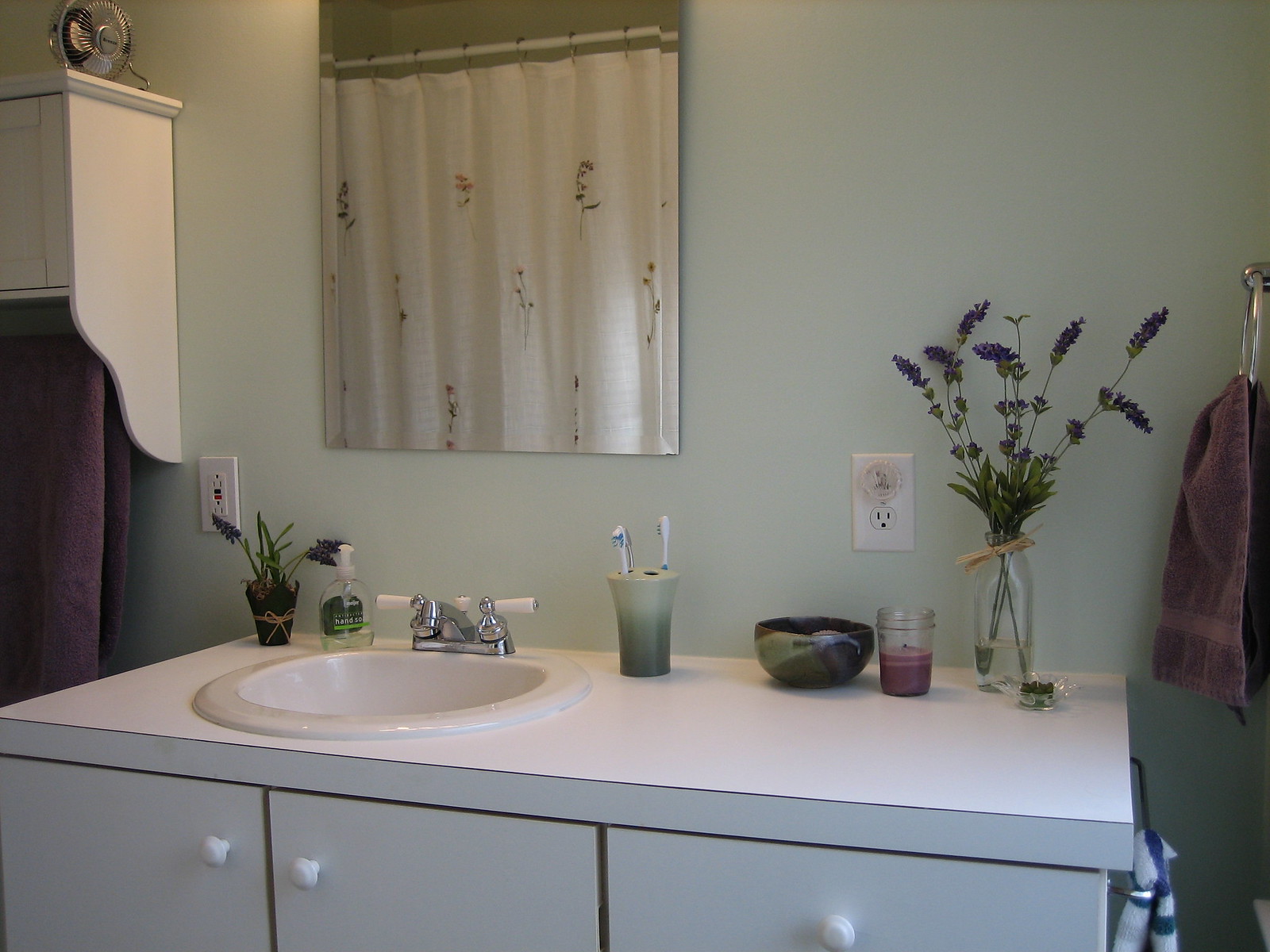This photograph showcases a well-maintained bathroom featuring a pristine white countertop. On the countertop, there is a neatly placed soap dispenser, adding a touch of practicality to the space. A charming flower vase, filled with fresh blooms, brings a pop of color and a natural aesthetic to the otherwise sleek and modern setting. The background reveals a portion of the bathroom mirror, which reflects a view of the shower curtain, contributing to the sense of depth and providing a wider glimpse into the room's decor. The overall scene exudes cleanliness and simple elegance.